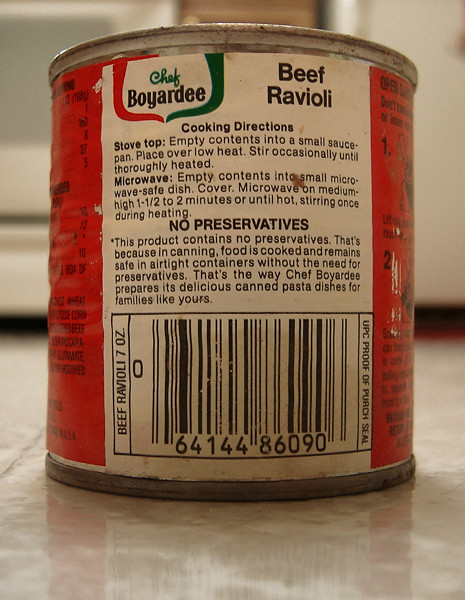The photograph showcases a vintage and heavily rusted can of Chef Boyardee Beef Ravioli, featuring an aged design indicative of its antique status. The label, adorned predominantly in white and red, occupies most of the can's surface. A prominent wide white rectangle centered on the label is flanked by red sections on either side. The "Chef Boyardee" logo is presented in various shades of green, with 'Chef' in a lighter green script and 'Boyardee' in a darker green. Bordering the logo are red on the left and dark green on the right, framing the description of "Beef Ravioli" in black text. Additionally, the label details cooking instructions for both stove top and microwave, highlights the absence of preservatives, and includes a barcode. The can's dimensions and appearance—traditional cylindrical shape, silver aluminum material, and significantly corroded—emphasize its weathered state. Positioned on what seems to be a reflective, white, and tan kitchen tile floor, the background of the image subtly reveals parts of an oven and refrigerator, implying a kitchen setting. The tile floor below, likely adorned with subtle floral patterns, reflects parts of the can, adding a contextual background to this evocative depiction of a culinary relic.